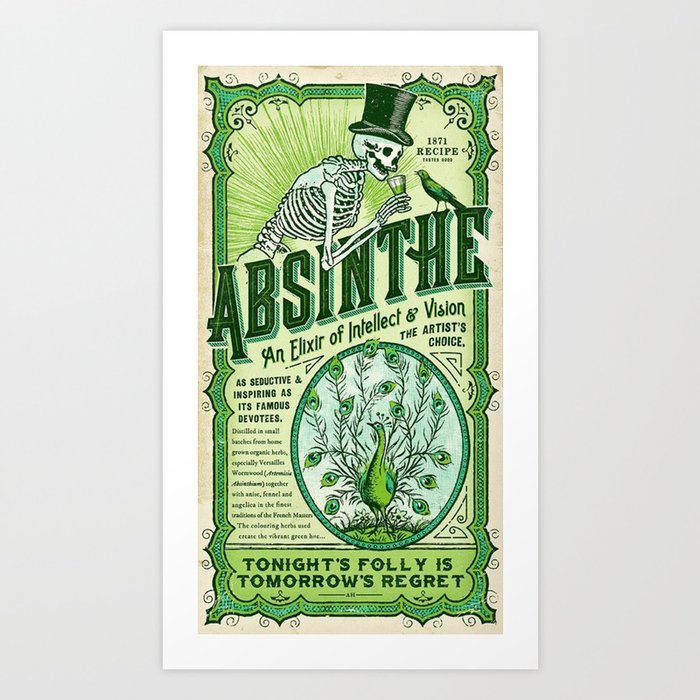This vertical rectangular artwork features a vintage-style label displayed against a gray background. In the center is a poster with a white border and predominantly green interior. At the top, a skeleton wearing a top hat is depicted drinking from a glass while a raven perches in front of him. Large, dark green letters spell out "Absinthe," followed by the tagline "An elixir of intellect and vision" in smaller green letters. Beneath this, it reads "The artist's choice" and "1871 recipe," along with the phrase "As seductive and inspiring as its famous devotees." The image also includes an ornate border and an illustration of a green peacock with its feathers fanned out. At the bottom, against a green background, the ominous warning "Tonight's folly is tomorrow's regret" is inscribed in darker green text. This intriguing composition resembles an advertisement for a historical absinthe beverage, blending artistic elements with a touch of whimsy and caution.